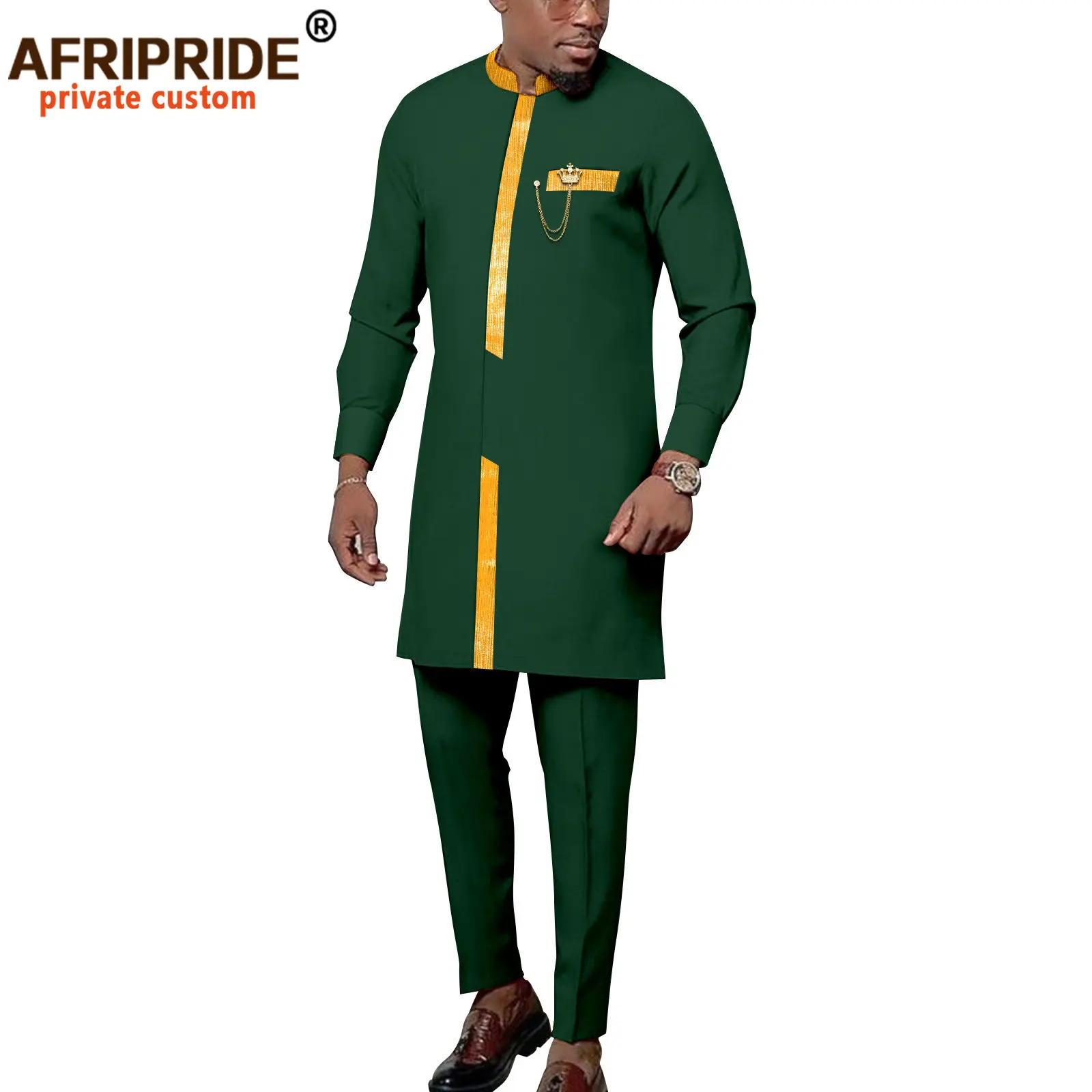In this advertisement with a plain white background, an African American gentleman is modeling an elegant, custom-designed outfit by AfriPride, prominently featuring its registered trademark and the tagline "Private Custom" in red text at the top left corner. The man is wearing a striking, forest green tunic that extends halfway down to his knees. This tunic is adorned with gold accents around the collar and features a distinctive yellow stripe that runs down the center, concludes midway, and then continues to the bottom. Complementing the tunic, he has on slim, forest green trousers and stylish brown loafers. His look is completed with a sophisticated wristwatch. The top half of his face is cut off in the image, emphasizing the detailed design and craftsmanship of the attire while suggesting a focus on the clothing's appeal for special occasions.